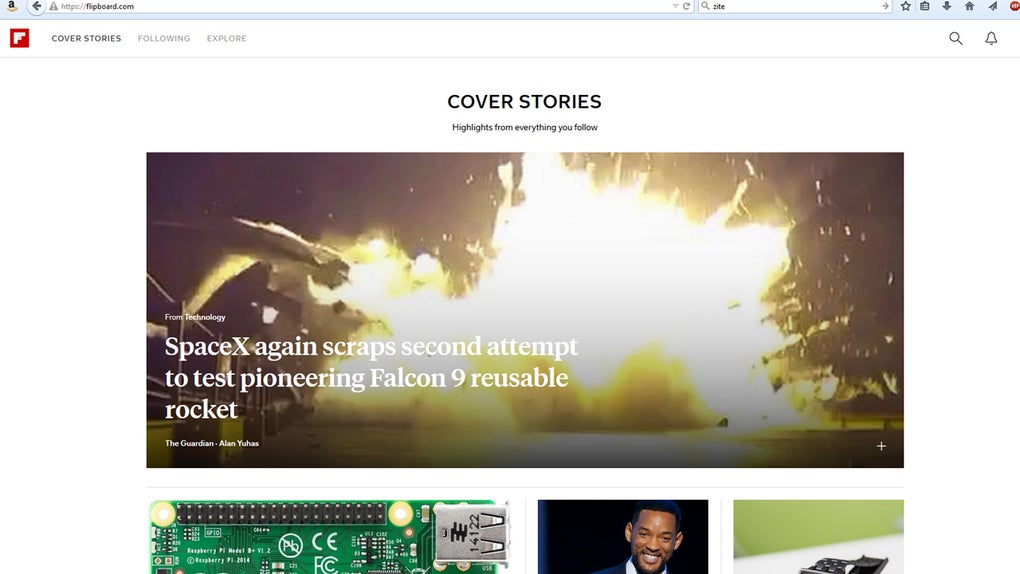This is a detailed screenshot of the website Flipboard (https://flipboard.com). The image captures the interface as seen on a classic Windows-themed browser.

At the very top, the address bar is clearly visible with the site's URL displayed. To the right of the address bar, there's a search bar with text input reading "DITE." Next to the search bar are several functional icons: a favorites star, a clipboard, a download button, a home button, an unidentified button showing a cursor, and a stop sign.

Beneath the browser's address bar, the Flipboard logo is prominently displayed. The logo consists of a white "F" inside a red square. Adjacent to the logo, the word "Cover Stories" appears, which is currently selected. Other navigation options include "Explore" and "Following." On the far right, icons of a magnifying glass (search) and a bell (notifications) are also visible.

In the main part of the screen, "Cover Stories" is highlighted in bold black capital letters, accompanied by the subtitle "Highlights from everything you follow." Below this heading, there is a featured image from a technology article titled "SpaceX again scraps second attempt to test pioneering Falcon 9 reusable rocket." The image depicts a bright yellowish explosion against a dark background, with NASA-related objects nearby. This article is credited to The Guardian and authored by Alan Hughes. The visual effects of the explosion dominate the scene with varying shades of yellow, ranging from bright to dark.

A thin gray line separates this main section from subsequent content. To the left, a small image displays what appears to be a computer USB port card. A vertical gray line divides this image from another segment featuring Will Smith grinning, set against a black rectangle. Further to the right, another gray vertical line separates this segment from an image of what seems to be a watch band, although the watch itself is off-screen.

This detailed screenshot encapsulates the organized yet dynamic layout of the Flipboard website, providing a glimpse into its user-friendly interface and content arrangement.